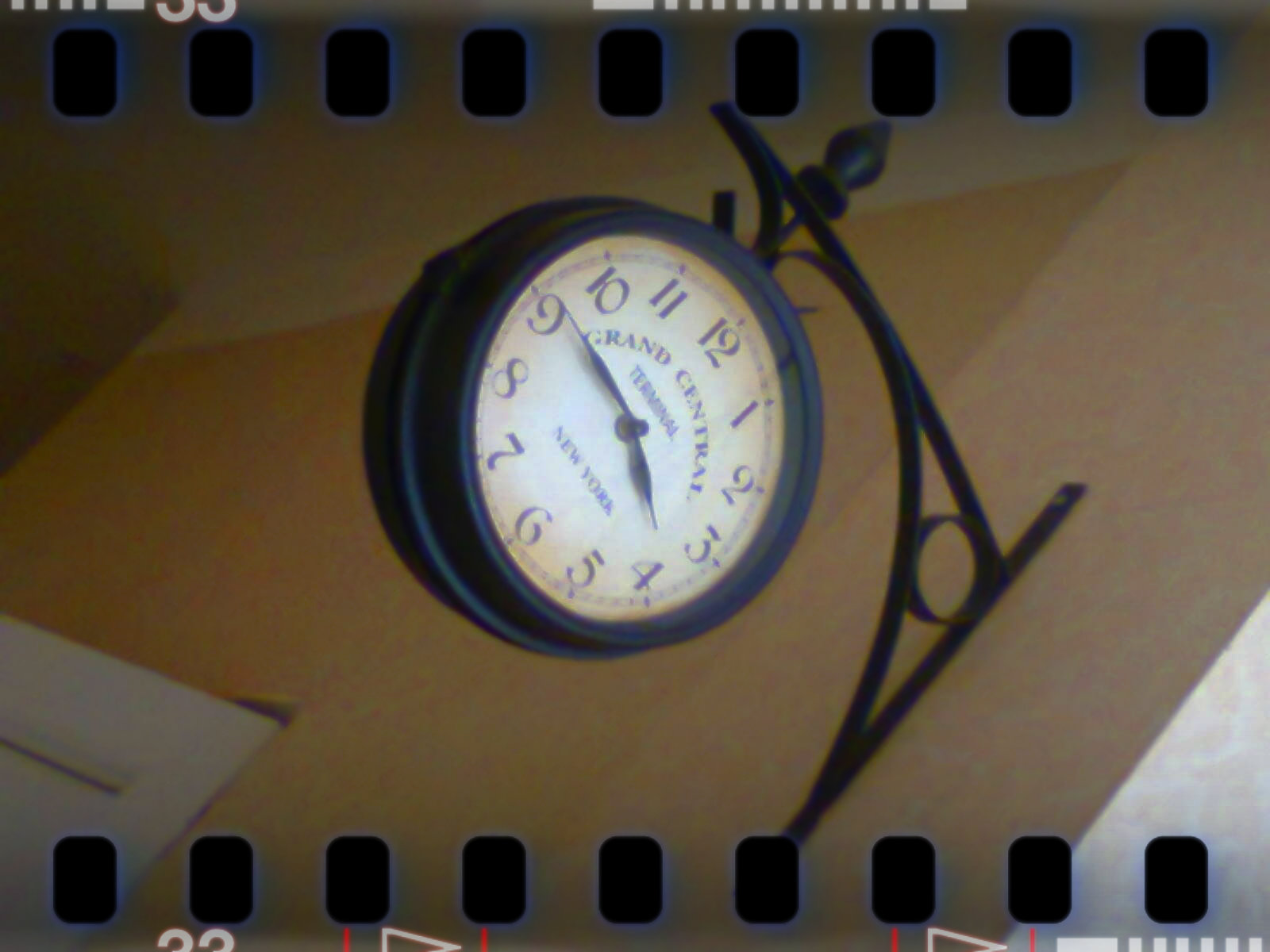The image appears to be a scan or an artistic overlay mimicking a film negative. The centerpiece is a vintage clock mounted to a wall with sleek black hardware. The clock face prominently displays the inscription "Grand Central Terminal New York." Adding to the nostalgic aesthetic, the image features a series of tiny black rectangles with rounded corners—a characteristic of film negatives—running as a stripe along both the top and bottom edges of the frame. This detail reinforces the impression that the photograph is captured or rendered in a style reminiscent of classic film photography.